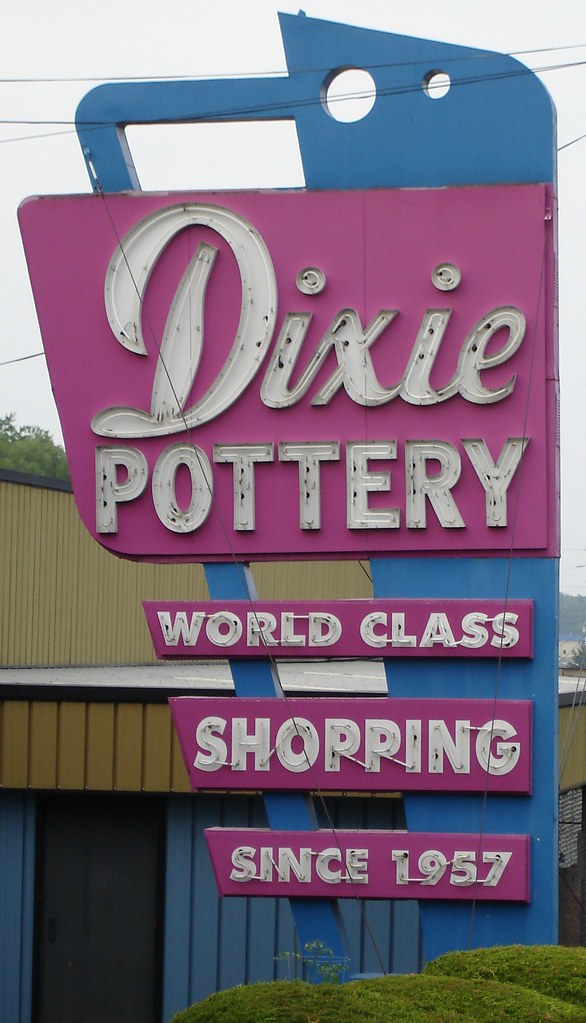The image depicts a vintage business sign with a distinct, aged appearance. The main portion of the sign is predominantly blue, and features a graphic resembling a hacksaw, slightly tilted and resting across the front, giving it a unique, nostalgic look. Attached to this central blue section, a larger pink sign prominently displays the name "Dixie Pottery" in bold letters. Below the main sign are three smaller, thin signs with white text. The first sign reads "World Class," the second says "Shopping," and the third boasts "Since 1957." The combination of colors and design elements gives the sign a classic, enduring charm.